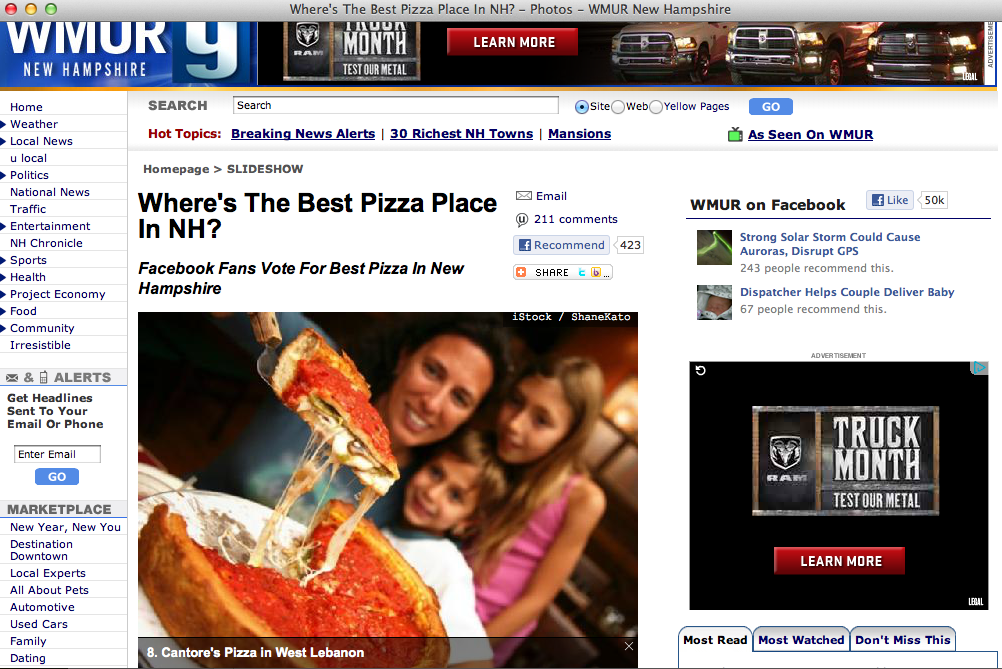This image depicts a webpage from WMUR9 in New Hampshire, featuring a detailed and vibrant layout. 

At the very top, a thin banner poses the question, "Where's the best pizza in NH?" suggesting an engaging local topic. Just below this banner sits an advertisement for Ram Trucks, promoting their "Truck of the Month" with the tagline "Test our metal, learn more." The ad features three gleaming trucks lined up side by side, enticing potential buyers.

On the left side of the webpage, there is a vertical menu with various selections, including Home, Weather, Local News, U Local, Politics, National News, Traffic, Entertainment, Sports, Health, Project Economy, Food, Country, Community, Irresistible, some alerts, and a Marketplace section. This navigation bar provides easy access to a wide range of information and services.

The center of the page highlights a homepage slideshow under the banner "Where's the best pizza in NH?" which invites Facebook fans to vote for the best pizza in New Hampshire. Dominating this section is a large, colorful photo featuring a woman and two children proudly presenting a sizeable, two-layered pizza. The caption identifies the pizza as Cantatori's Pizza from West Lebanon.

On the right side, there is another advertisement for Dodge Truck Month, ensuring that the promotion catches the viewer’s eye from multiple angles on the webpage. 

Overall, the page combines local interests with targeted advertising, creating a dynamic and user-friendly interface.